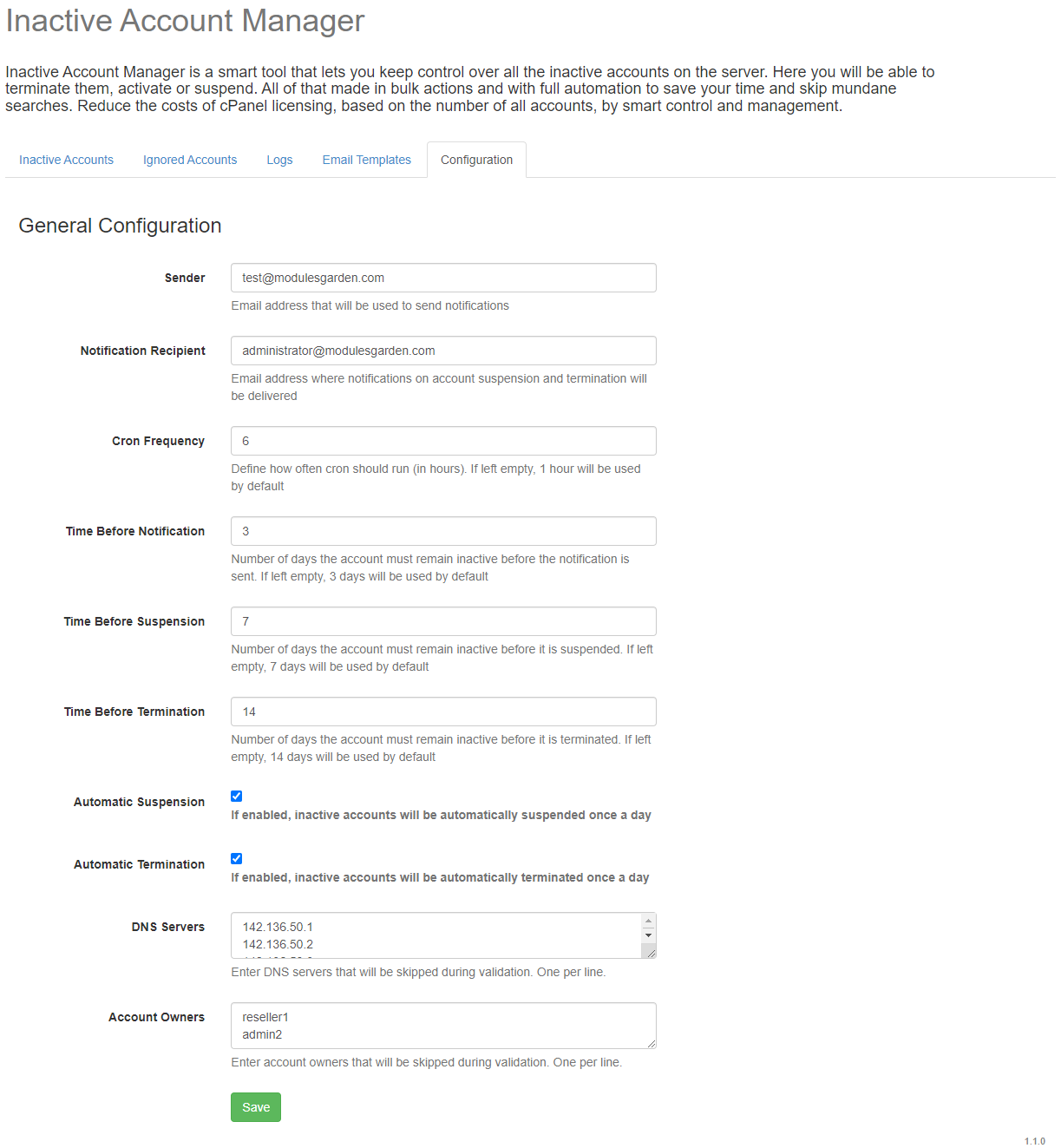This image is a detailed screenshot of a website interface for managing inactive accounts. At the top left corner, the heading "Inactive Account Manager" is displayed in grey text. Directly below it, there is a smaller black text description which reads: "Inactive Account Manager is a smart tool that lets you keep control over all the inactive accounts on the server. Here you'll be able to terminate, activate, or suspend them. All of that made in bulk actions and with full automation to save your time and skip mundane searches. Reduce the cost of cPanel licensing based on the number of all accounts by smart control and management."

Below this description, several tabs are lined up from left to right: "Inactive Accounts," "Ignored Accounts," "Logs," "Email Templates," and "Configuration." 

On the left-hand side under the "Configuration" tab, an additional heading “General Configuration” is visible. Below this are several entry fields for various settings: "Sender," "Notification Recipient," "Cron Frequency," "Time Before Notification," "Time Before Suspension," "Time Before Termination," "Automatic Suspension," and "Automatic Termination." There is also a section for entering DNS servers with two servers already listed. Further down, there is an "Account Owners" section showing two entries: "Reseller 1" and "Admin 2." At the bottom of the page, there is a prominent green "Save" button.